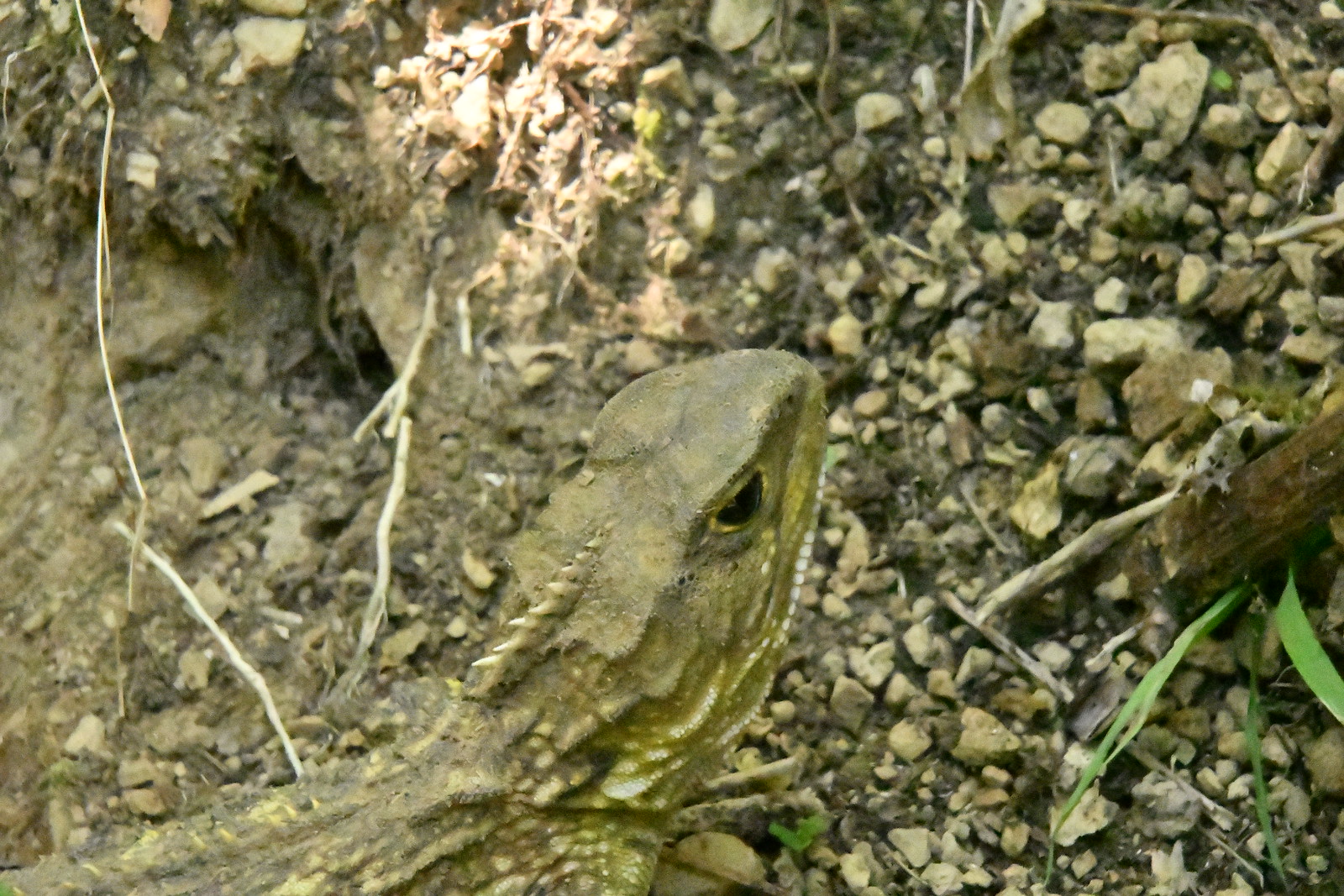This daytime photograph captures a partially visible iguana, with just its head and part of its upper body in view, located at the bottom left corner of the image. The iguana is positioned amidst a terrain of loose gravel, dirt, and protruding plant roots. A subtle gradation of the image lighting, brighter at the top due to sunlight, hints at the outdoor setting. The ground features a few blades of green grass in the bottom right corner. The iguana exhibits a palette of greens, ranging from dark to light, accented with white spots. Its most striking feature is a white spiked dorsal fin that runs along its spine from the head. The iguana’s black eye faces the top right of the photograph, giving it an attentive look as it appears to blend seamlessly with its earthy surroundings.